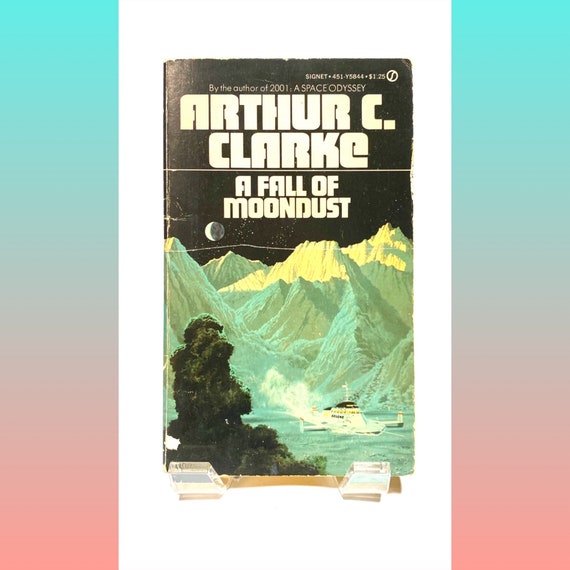This is a square image with a gradient background transitioning from a blue-teal at the top to a dark pink at the bottom. Centered within this backdrop is a vertical white rectangle, inside which is a photograph of an old, weathered paperback book cover. The cover is predominantly black and exhibits signs of age with bends and cracks. At the very top of the cover, small white text reads "Signet 451YS844, $1.25." Below, in larger white letters, it states "by the author of 2001, A Space Odyssey," followed by "Arthur C. Clarke" in the largest font, and "A Fall of Moondust" underneath.

The book cover's image consists of a moon with stars against a dark sky. Below this, a series of white, spiky mountains sit against a greenish-yellow landscape. At the bottom of the cover, a large white craft, possibly a space station or vehicle, lies amidst white smoke or fog. In the foreground, a dark green, possibly vegetative mass or creature with a discernible face adds a mysterious element to the scene. The edges of the book appear tattered, emphasizing its age and long history.